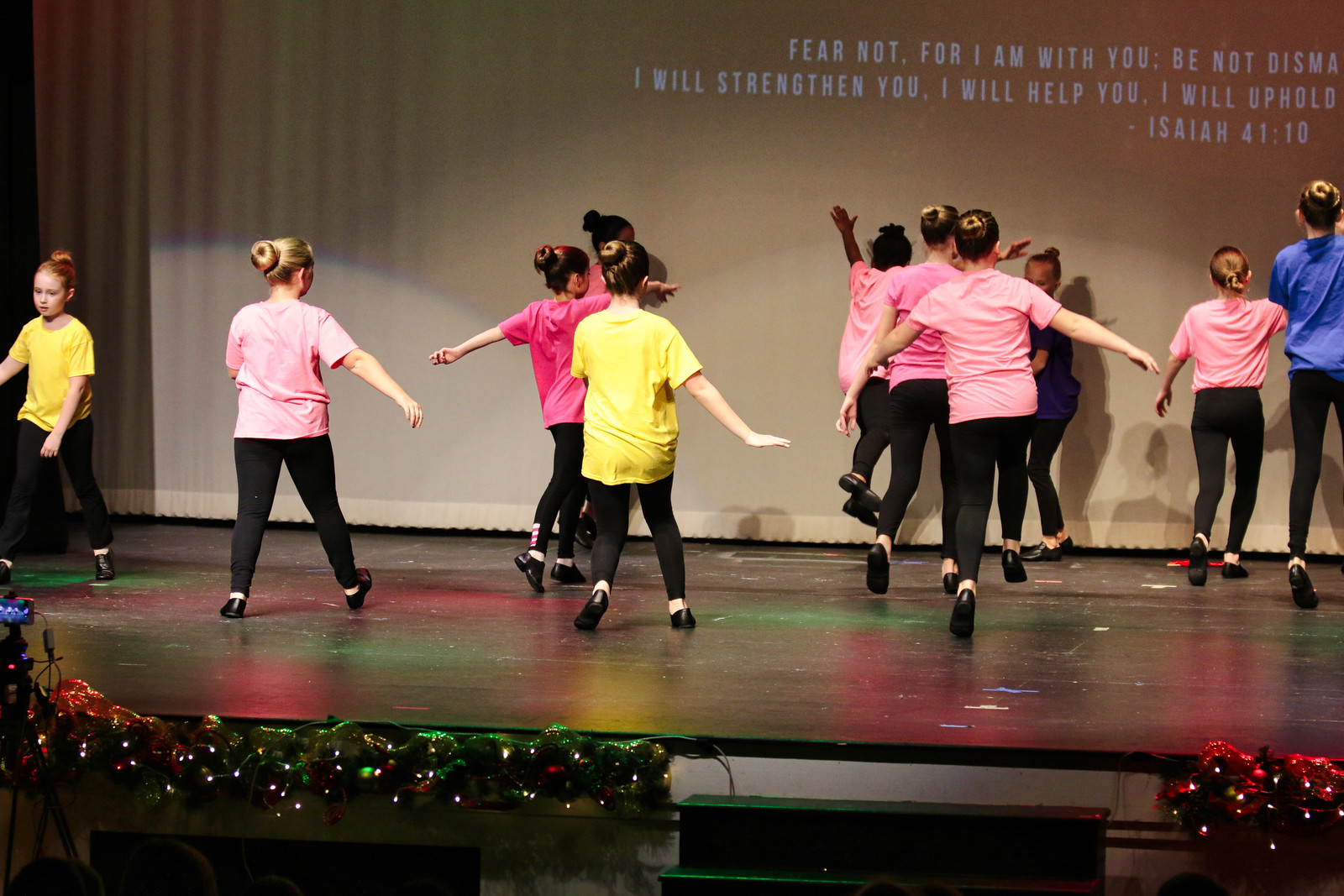The horizontal rectangular image captures a group of young children, likely all girls, ranging in age from about 6 to possibly 14, performing a dance routine on a dark brown stage. The stage is adorned with Christmas decorations, including holly and lights, especially at the front. Two staircases leading up to the stage are visible. The dancers are all dressed in black pants and black shoes, with their bare heels showing. They sport colorful T-shirts in shades of pink, yellow, and blue. Most of the children have their backs to the audience, except for a young girl on the far left, who has red hair and is wearing a yellow shirt. The background features a beige-colored wall and a screen displaying a Bible verse in white letters: "Fear not, for I am with you; do not be dismayed, I will strengthen you, I will help you, I will uphold you," from Isaiah 41:10. The children are in various positions corresponding to their dance steps, with many having their arms spread out. There are no audience members visible in the image. The setting suggests a festive dance performance, possibly as part of a Christmas celebration at a church or a public venue.